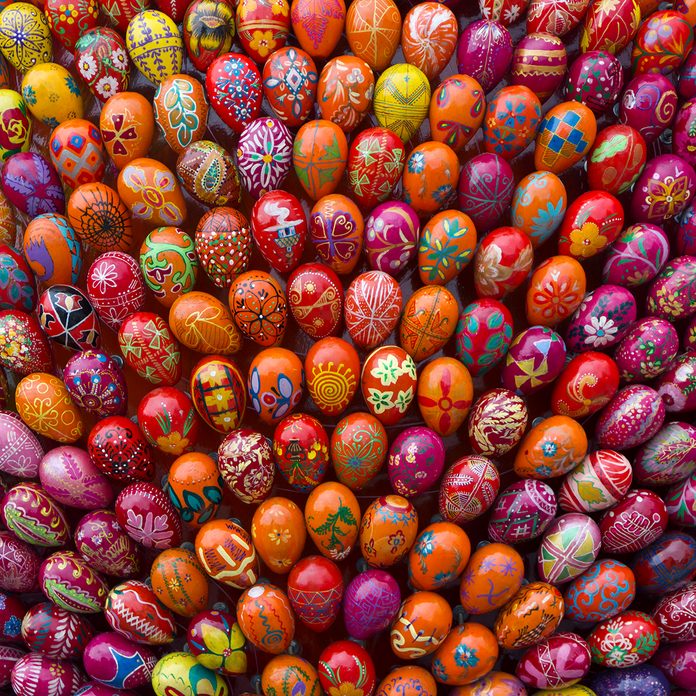This vertical rectangular image showcases an up-close view of over a hundred meticulously painted Easter eggs, arranged in a visually striking pattern resembling the spokes of a wheel. Each egg is adorned with intricate designs in a vibrant array of colors, including prominent shades of orange, pink, purple, blue, yellow, red, turquoise, green, and white. The eggs are placed in semi-circular concentric circles, originating from a central point at the bottom. In the foreground, there are three eggs in an arc, followed by successive layers, each increasing in number as they radiate outward, creating a solid, colorful display. The designs include detailed motifs such as butterflies with red and purple wings and intricate gold heart shapes, flowers with red petals and gold centers, and various leaf figures. The overall pattern and design are dense and mesmerizing, making for a rich and engaging visual experience.